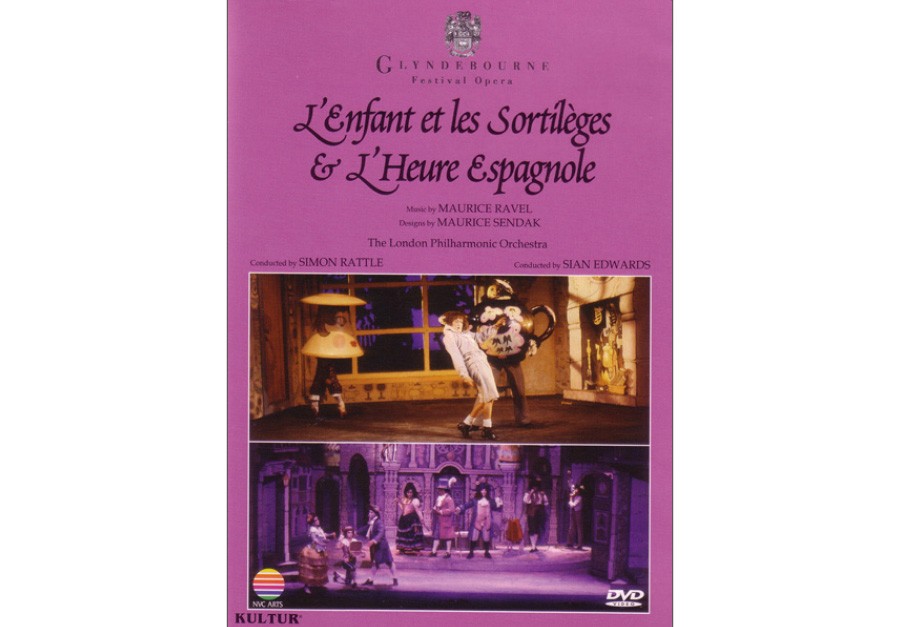This vertically aligned rectangular image, which appears to be a DVD cover, features a vibrant purple-pink background at the top. It prominently advertises the Glyndebourne Festival Opera. In larger black print, it highlights the performances of "L'Enfant et les Sortilèges" and "L'Heure Espagnole." The music is composed by Maurice Ravel, with designs by Maurice Sendak. The left side lists Simon Rattle as a conductor, and the right side lists Sian Edwards. 

The bottom section of the cover is taken up by two horizontally aligned, rectangular photographs depicting scenes from the opera. The first image shows a slightly blurry performance with a person on stage in front of a window and two other costumed characters. The second image portrays several characters lined up on a darker stage, engaging in a performance. The lower right corner of the cover indicates "DVD," and the lower left corner features the text "Kultur."